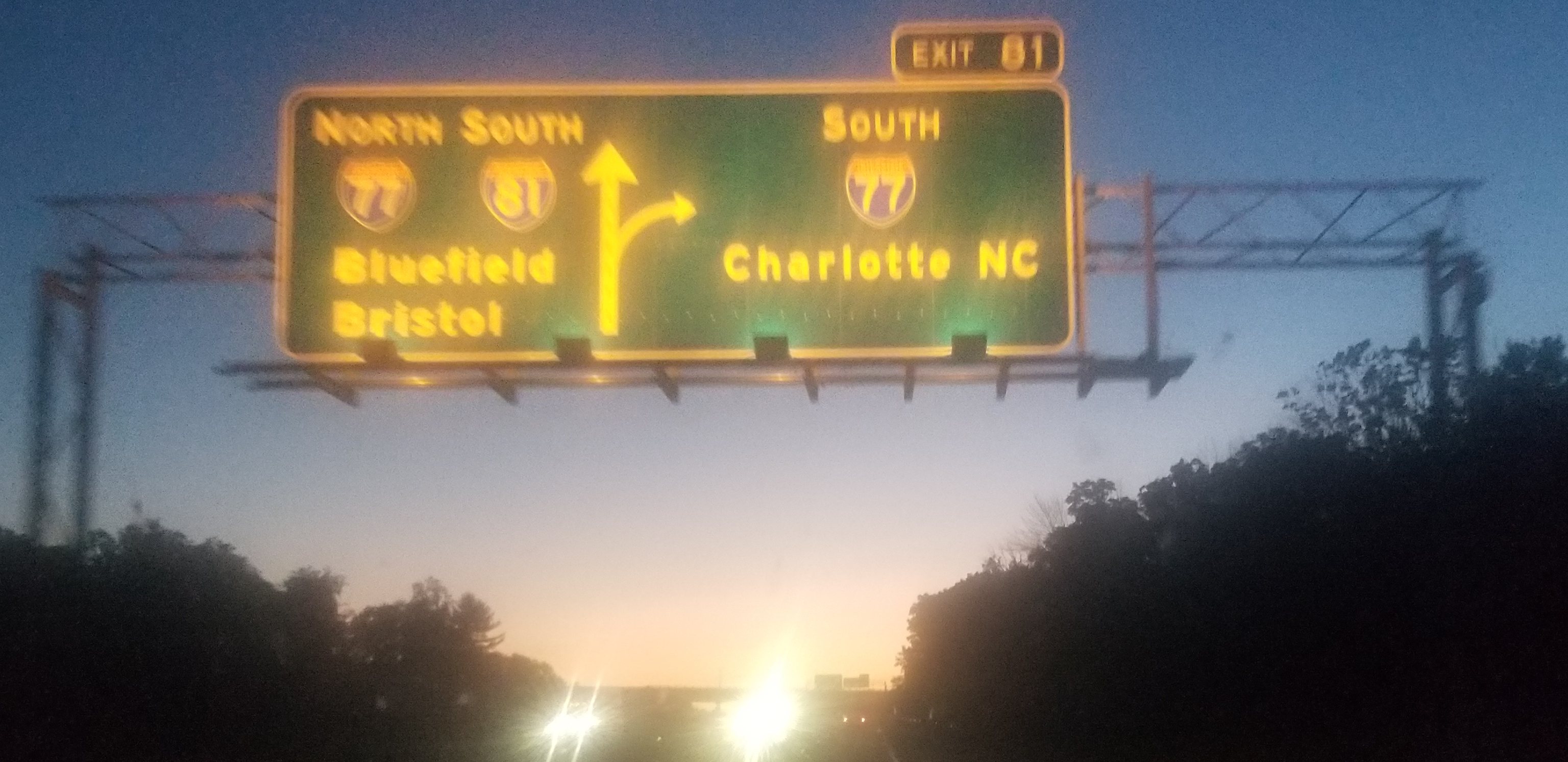This image captures an overhead road sign mounted on an expressway, supported by steel poles on either side. The structure holds a prominent green sign with a smaller banner positioned in the top right corner from the camera's perspective. The top smaller sign is green with a white border, displaying "Exit 81" in white characters. Below it, the large green sign with a white border features directional information.

The sign reads "North" and "South" in white letters, indicating interstate highways and destinations. "North 77" is presented within a white-lettered red and blue shield. "South 77" also appears within a similar white-lettered shield. "South 81," positioned over the southbound indication, is marked within a white-lettered shield as well. Arrows point straight ahead for "North 77" and "South 81," directing travelers to Bluefield and Bristol. An arrow points right for "South 77," leading towards Charleston, North Carolina.

The expressway is lined with trees on either side, and the image captures a serene evening sky, painted with light blue, pink, and white hues at the horizon. Bright headlights of oncoming traffic are visible at the bottom of the image, enhancing the urban ambiance.